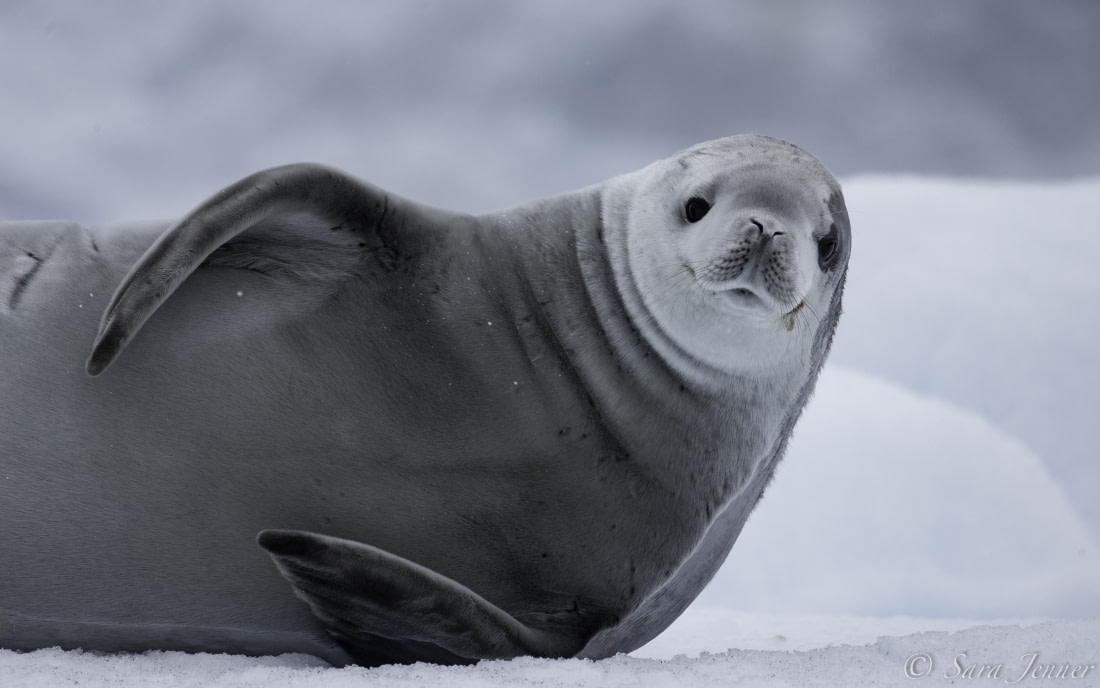In this captivating black and white photograph by Sarah Jenner, a seal is prominently featured in the foreground of an Arctic landscape blanketed in snow. The background, though slightly blurry, hints at a cold and snowy region with a cloudy gray sky. The seal, leaning into the frame from the left side, is depicted in a relaxed yet alert pose as it lies on an icy surface. Its head, positioned about a quarter of the way from the right edge of the image, is light gray with whiskers clearly visible on its muzzle. The seal's face and neck are white, contrasting with its smooth, shiny black belly and flippers. Its top head area is a smoky gray, matching the gradual darkening of the body from the head down. The seal's curious eyes meet the camera directly, giving it a friendly and engaging expression. The overall scene is a serene and detailed portrayal of the seal in its natural, frosty habitat, beautifully captured by the photographer.